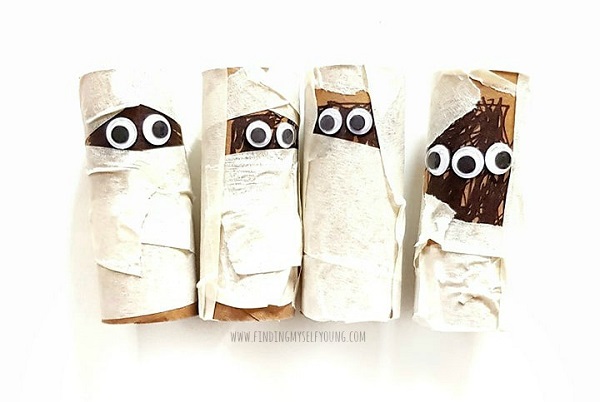This image showcases an art project, potentially created by a child, featuring a row of four empty toilet paper rolls arranged to resemble small mummies or ghosts. Each roll is meticulously wrapped in white tissue, with the tops of the rolls shaded in dark brown marker to simulate faces. The most striking feature is the googly eyes of various counts, glued onto each roll, with three eyes on one roll for a unique touch. Set against a plain white background, the rolls are predominantly brown and white in color. The project is underscored by the website www.findingmyselfyoung.com displayed below the art pieces.